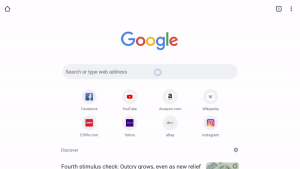The image depicts a Google homepage. In the top left corner, there is a home page icon, while the top right corner contains a file icon and an ellipsis (three-dot) menu icon. Dominating the center is the iconic Google logo, featuring the blue capital 'G,' red 'O,' yellow 'O,' blue lowercase 'g,' green 'l,' and red lowercase 'e.' Below the logo is the search bar, prompting users to "search or type web address."

Under the search bar, there is a row of frequently visited website icons: 
- Facebook icon, accompanied by the text "Facebook."
- YouTube icon, accompanied by the text "YouTube."
- Amazon icon and text "Amazon."
- An unidentified icon that is too blurry to recognize.
- An icon featuring a red square in the middle, situated at the bottom left of the row.
- Yahoo icon, followed by the text "Yahoo."
- eBay icon, with the text "eBay."
- Instagram icon, and next to it, the phrase "fourth stimulus check, even add new relief."

This detailed layout illustrates a typical web browser start page with quick links to popular websites.